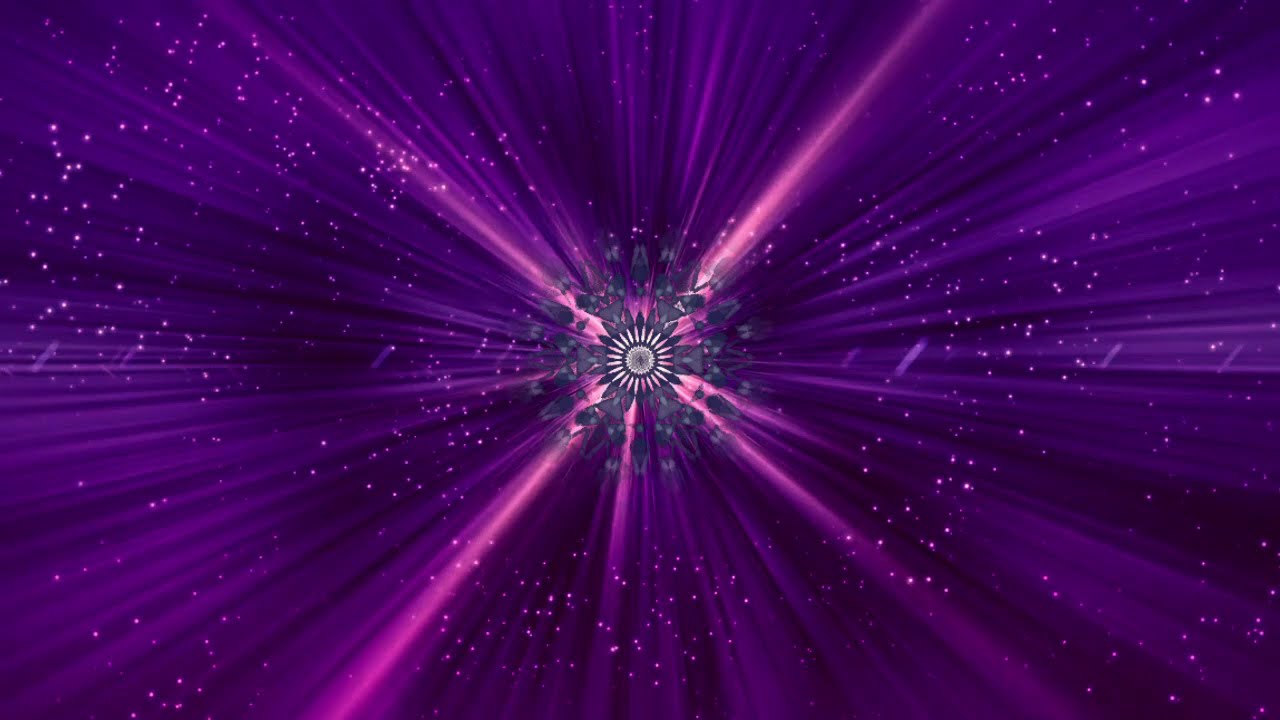The image depicts a mesmerizing purple burst of light creating radiant rays against a dark night sky scattered with white specks resembling stars. Central to the composition is a geometric, kaleidoscope-like pattern in shades of dark blue, gray, and white. This intricate, symmetrical design evokes the appearance of a spinning wheel or gear, possibly in motion, as if breaking apart into black and gray shards. Radiating from this center are vibrant streaks of magenta, pink, and various shades of purple, giving the impression of a dynamic explosion of color and light. The background enhances the celestial theme with its dark, starlit expanse, reminiscent of a vintage Windows screensaver or a cosmic journey depicted in a comic. The overall effect is a stunning blend of sparkling starlight and dynamic motion, creating a vivid and immersive visual experience.